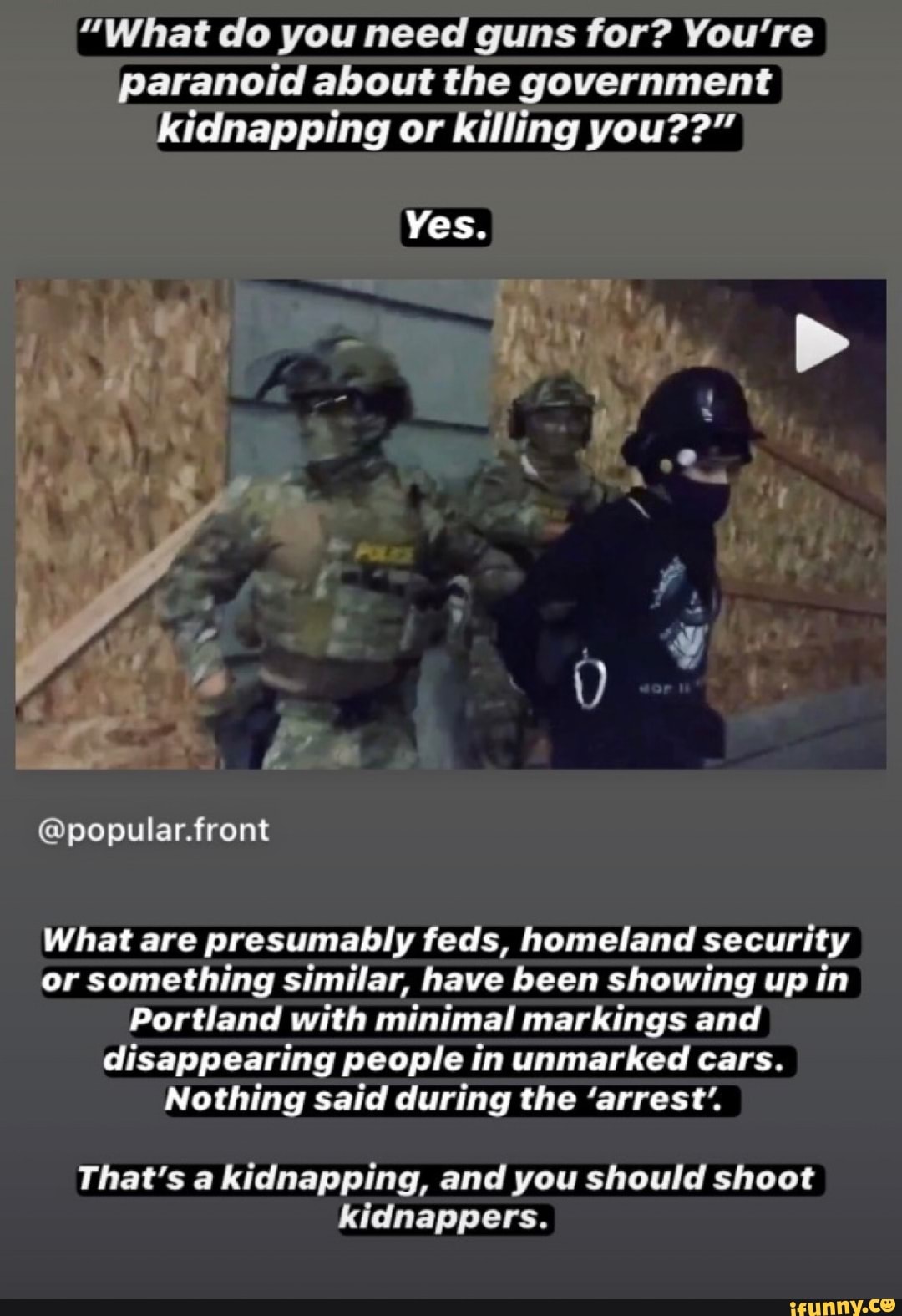A grainy photograph is bordered by dark gray bands at the top and bottom. The central image depicts two individuals outfitted in green army fatigues and bulletproof vests labeled 'POLICE'. They are wearing riot helmets and are handcuffing a person dressed in a long-sleeved black shirt with a design on the front, along with a black helmet and a mask obscuring their face. In the top right corner of the photo, there is a white play button icon. The caption at the top of the image reads, "What do you need guns for, you're paranoid about the government kidnapping or killing you?" Below this, a smaller text simply states, "Yes." The bottom portion of the image explains further, "Presumably feds or Homeland Security agents have been appearing in Portland with minimal identification, detaining individuals, and using unmarked vehicles."